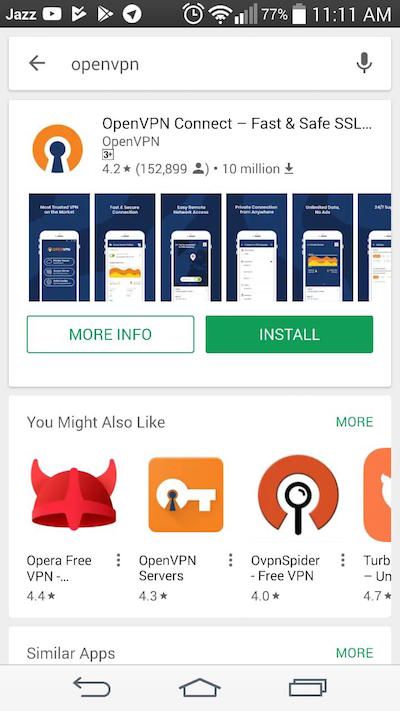In this detailed screenshot of an Android phone's app store, the screen captures the current status and search results at 11 AM. The battery level is at 77%, the phone signal strength is at two out of five bars, and the Wi-Fi signal strength is robust with four bars. An alarm clock icon is also visible. On the top left corner, the word "Jazz" is displayed, possibly indicating the carrier or a themed setting. To the right of "Jazz," there is a YouTube icon, a Google Play button icon, and two additional icons that are not clearly identifiable.

Centered below the status bar is a search bar containing the text "OpenVPN," indicating a search for VPN applications. To the left of the search bar is a back arrow, while a microphone icon sits on the far right, allowing for voice search. The primary search result presented is "OpenVPN Connect – Fast & Safe SSL," which boasts a 4.2-star rating based on 152,899 reviews and has achieved 10 million downloads. Accompanying the search result are images showcasing the app in use, along with two buttons: "More Info" on the left and "Install" on the right, providing options for the user to learn more about the app or to download it directly.